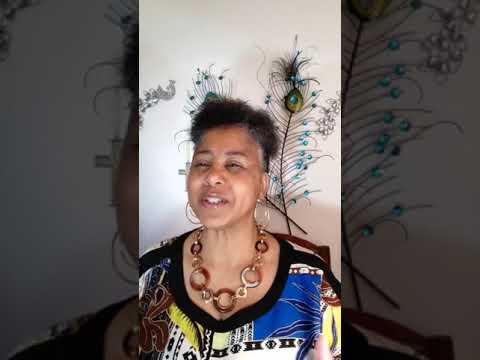The image is a composite photograph divided into three horizontal rectangles. The left and right rectangles display darker, partial views of the larger complete image. Both darkened side panels feature glimpses of a woman's face and a decorative feather that emerges from the bottom in the left panel and from the right edge in the right panel. The central rectangle, which is lighter and offers greater clarity, shows an older woman, possibly in her 50s, with a medium complexion and short, slightly graying brown hair. She is smiling and appears to be singing or speaking. She is adorned with large hoop earrings and an elaborate necklace of circular loops. She wears a multicolored shirt with a black collar, featuring hues such as blue, yellow, and white. Behind her, on a cream or light-colored wall, is an artistic decoration that resembles a feather or possibly a bird’s tail with beaded embellishments. The central panel presents the entire scene in full detail, creating a harmonious contrast with the darker, fragmented views on the sides.